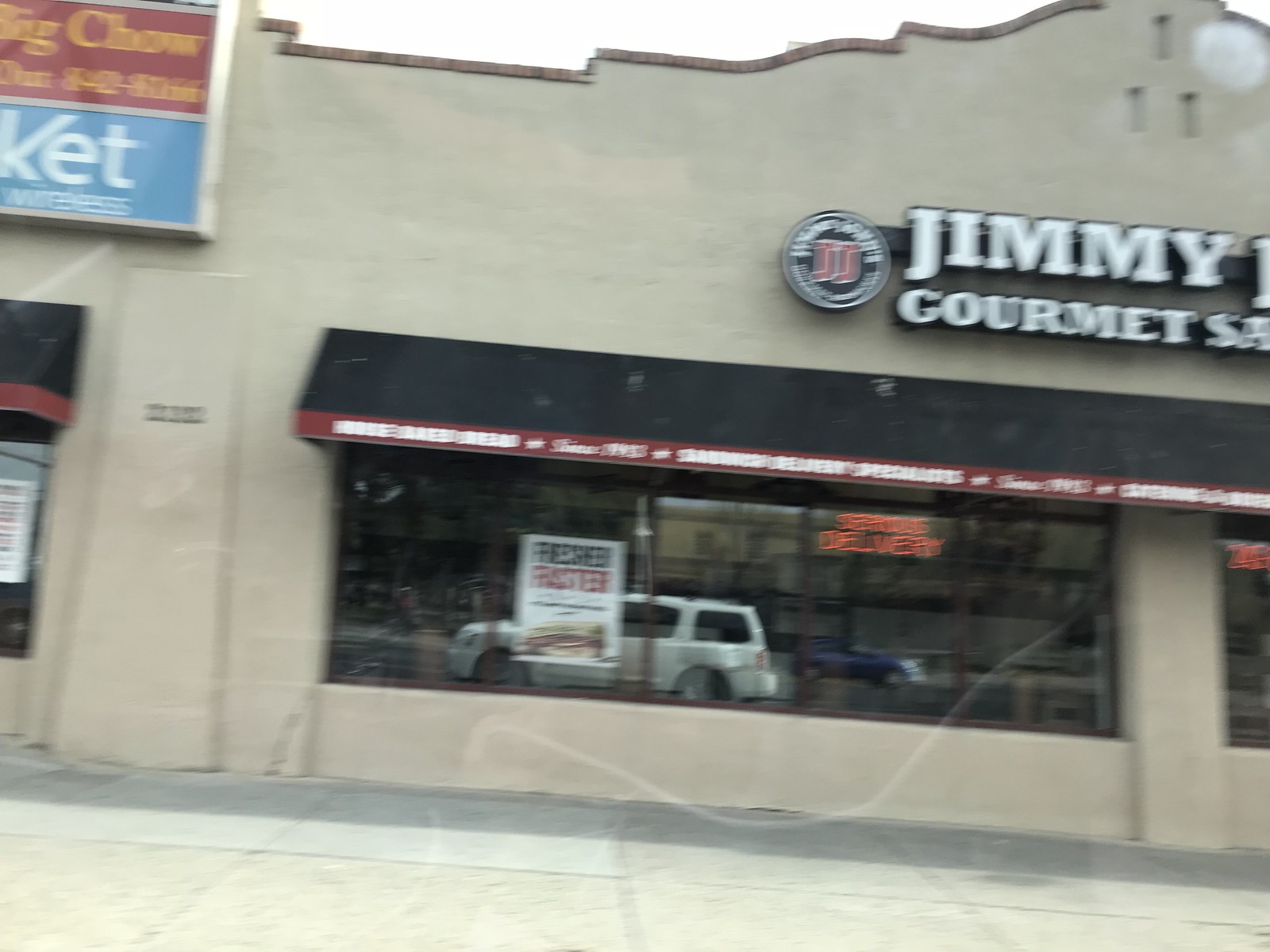The image depicts a beige, single-story storefront building with a darker brown trim. The photograph appears slightly blurred. Dominating the facade is a large picture window that spans the length of the building. Above this window, there's a dark black canopy. Higher up, above the canopy, the name "Jimmy Gourmet" is prominently displayed with the letters "JJ" encircled beside it. To the left of the main sign, another sign reads "Big Chow, K-E-T." A white truck is visible, its reflection captured in the large window at the front.